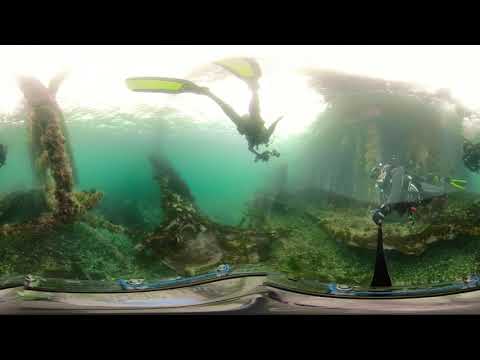The underwater image captures a group of scuba divers exploring a vibrant aquatic landscape. At the center, a diver with yellow fins is prominently holding a large camera, suggesting an intent to document the marine scene. Next to him, another diver, also equipped with yellow fins, is extending a selfie stick, creating a slight distortion indicative of a 360-degree panoramic shot. Further back to the right, another diver's face and goggles are visible, though their specific actions remain unclear due to the distance.

The divers are positioned near an underwater structure, possibly composed of rocks or pillars, adding a distinct geographical feature to the scene. On the left side of the image, various aquatic plants and mosses decorate the ocean floor, contributing to the biodiversity of the environment. The water itself is a clear yet slightly murky turquoise-blue, indicating good visibility with sunlight creating a reflective white sheen at the surface. Overall, the bright midday light enhances the vivid colors in the image, making the blues, greens, and yellows pop against the underwater expanse.